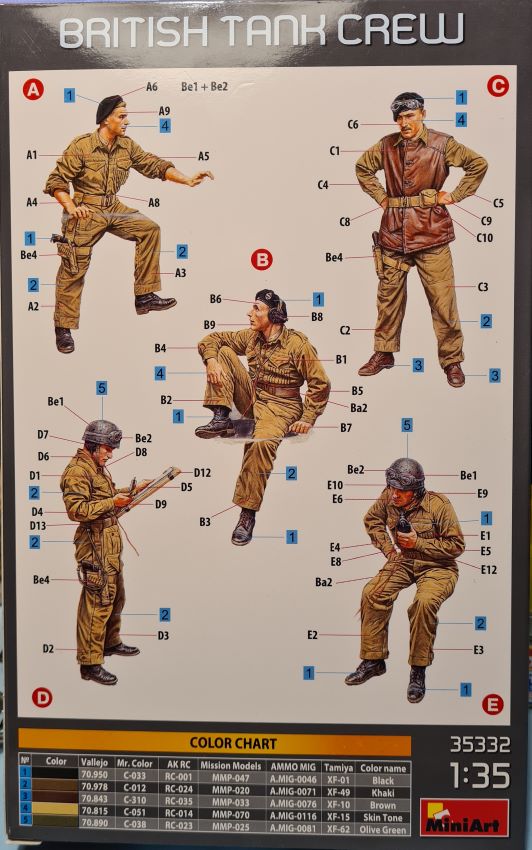The image features an order form from a magazine showcasing a detailed scale model kit named "British Tank Crew." At the top, the title "British Tank Crew" is prominently displayed. The center of the image presents five photographs of a figure dressed in a detailed military uniform. Various numbers annotate different parts of the uniform, including the helmet, badges, pockets, and various other areas, presumably pointing out specific features or colors.

In the bottom right corner, the code "35332" is printed, followed by the scale "1:35," indicating the model's dimensions. Additionally, there is a red rectangle with the brand name "Mini Art" written in black text.

To the left, the section titled "Color Chart" is illustrated with a table. The table has multiple columns, with the first column listing the numbers 1 through 5. The second column is labeled "Color" and includes hues such as brown and yellow. Subsequent columns provide corresponding paint brands: Vallejo, Mr. Color, AKRC, Mission Models, Ammo Mig, and Tamiya. The final column, "Color Name," lists the paint colors: black, khaki brown, skin tone, and olive green.